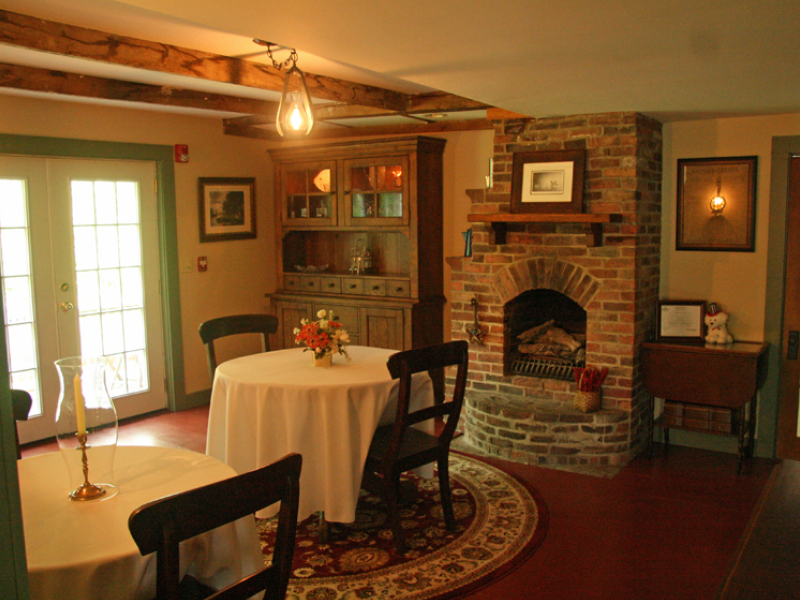The photograph captures a warm and cozy interior, possibly of an antique New England-style restaurant or an old-timey cottage-turned-establishment. The room is bathed in soft lighting accentuated by a small hanging lantern. The wooden ceiling beams lend a rustic charm, while a brick fireplace sits gracefully on a cream-colored wall. Two tables, each adorned with white tablecloths, are set intimately with just two wooden chairs per table, evoking a sense of coziness perhaps suited for a speed dating event or a quiet meal. One table features a candle in a glass vase, and the other an elegant basket of flowers. The hardwood cherry floor is complemented by a round ornate rug beneath one of the tables. A green-bordered set of double glass doors allows for natural light to softly filter into the room, enhancing its charm. Modern touches mingle with the vintage ambiance, such as a fire alarm on the wall and a well-maintained wooden beam running across the ceiling. Additionally, a cabinet organizer adds to the room's functional yet homey feel, completing this elegant and inviting scene.